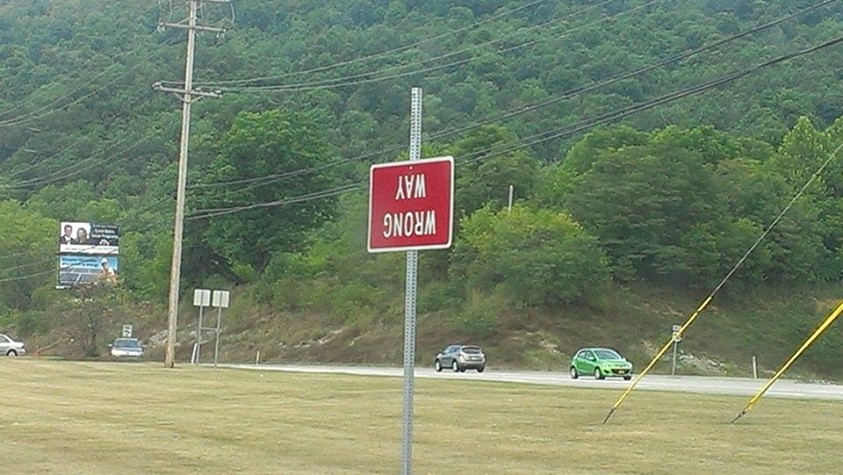In this image, a roadway stretches into the distance, with two cars prominently positioned near the center lower portion of the frame. A thick, hilly forest with dense rows of trees creates a lush, green backdrop, giving the scene a tranquil, forested ambiance. In the immediate foreground, a red "Wrong Way" sign is conspicuously placed, but oddly, it is upside down, attached to a square-shaped pole. To the left of the frame, a few billboards are visible, adding some urban elements to the otherwise natural setting.